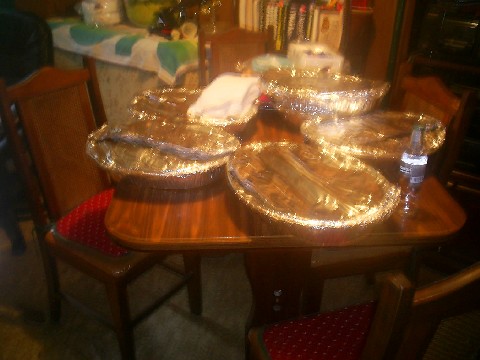A blurry photograph depicting a cozy, somewhat cluttered dining space, likely in a kitchen, illuminated by soft yellow lighting. Central to the image is a small, square wooden table with rounded corners. The table is surrounded by four matching wooden chairs, each featuring a cane back and red upholstered seats adorned with white polka dots and a green border. On top of the table, there are five large, oval-shaped platters with deep wells, all covered in aluminum foil. One of the platters on the back left has a white cloth resting atop it. Additionally, there's a bottle, possibly a beer, located at the bottom right of the table. In the background, various household items create a sense of lived-in clutter, including a row of books—potentially cookbooks—a towel on a bench top, and several kitchen appliances. An office chair is faintly visible on the far left, adding to the eclectic mix of items in the scene.